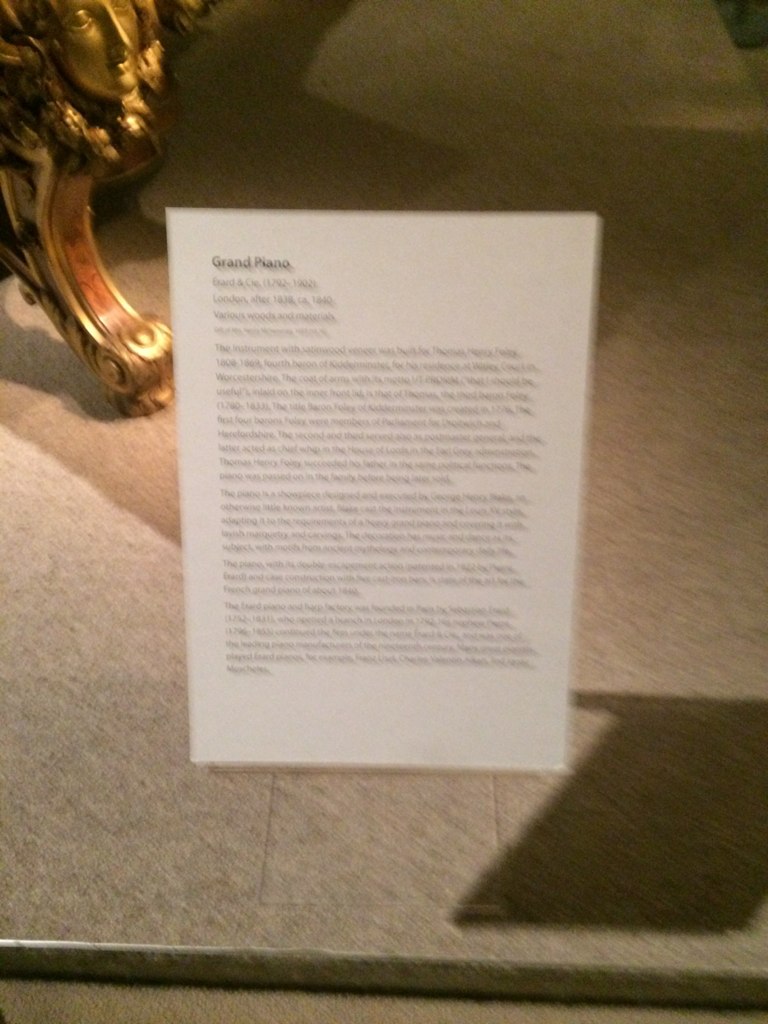The image captures a slightly blurry photo of a rectangular sheet of paper, appearing to contain a detailed description of a grand piano. The text on the paper is largely illegible due to the blurriness, but the top left corner prominently features the bold black words "Grand Piano." The paper is filled with three paragraphs of text, presumably containing intricate details about the piano. 

In the background, partially visible through the translucent quality of the paper, there appears to be a golden metal leg adorned with elaborate designs, which might belong to the grand piano being described. The image also includes a gray, somewhat nondescript ground surface. Overall, the main focus of the photograph is the descriptive paper that draws attention with its bold heading and substantial blocks of text, despite the blurriness that obscures the finer details.